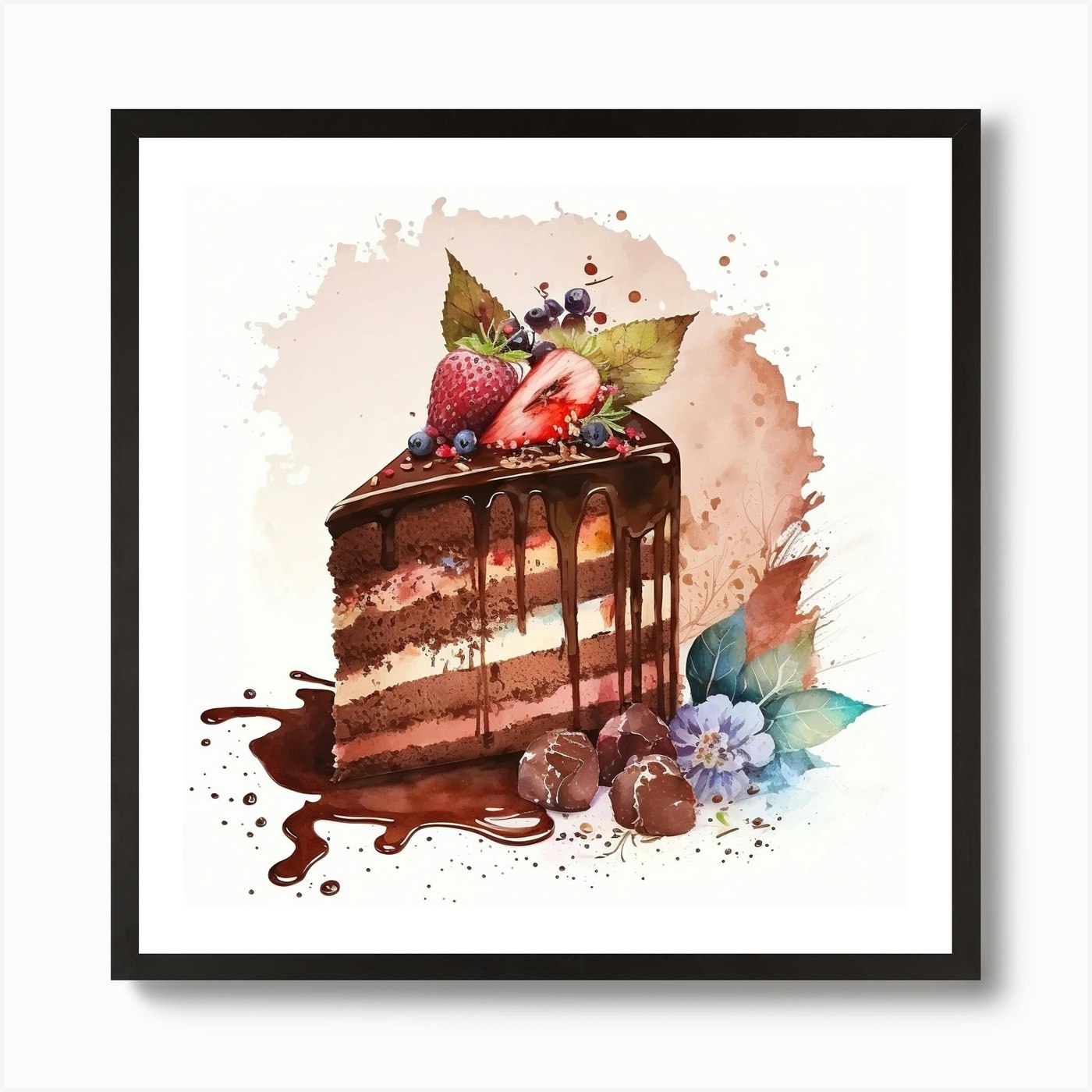The image is a black-framed picture displayed against a white background. The centerpiece is a multi-layered chocolate cake slice adorned with various elements. The cake boasts seven layers alternating between brown (chocolate), pinkish, and white fillings. Rich chocolate icing cascades down the sides, pooling at the base, creating a luscious effect. Atop the cake, there are strawberries— one sliced —alongside blueberries, adding vibrant colors and freshness. An intricate arrangement of garnishes includes a purple (or blue) flower to the right and three chocolate bonbons to the left of the flower, enhancing the visual appeal with their detailed positioning. The background subtly features a gradient of light pink to darker pink splotches, complementing the intricate presentation of the delectable treat in the foreground.